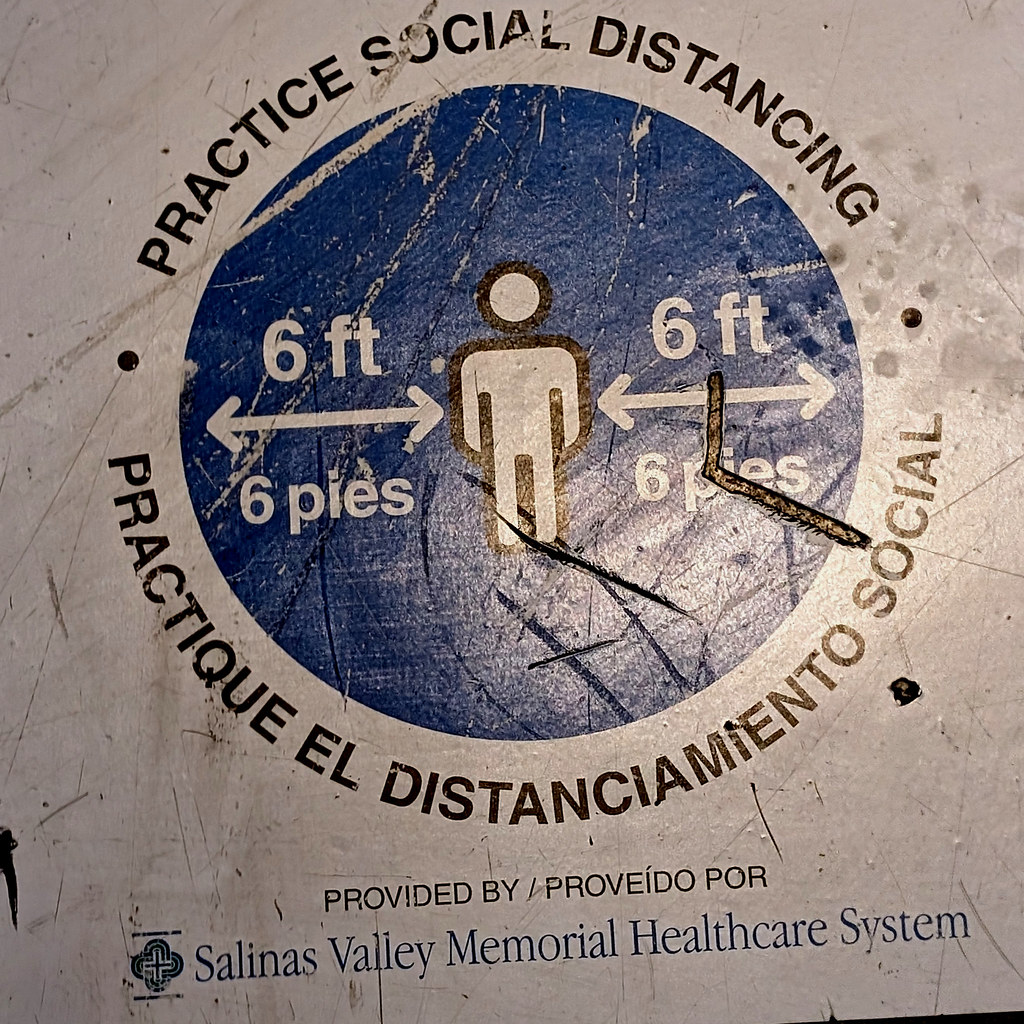The image features a solid white wall with a prominent, centrally-placed public service announcement. At the top, large black text reads "Practice Social Distancing," encircling a blue circle that contains a stick figure flanked by arrows pointing outward to indicate a distance of six feet. The same instructions are repeated in Spanish: "Practique el distanciamiento social," with the measurements "six feet" and "six pies" noted on both sides of the stick figure. Below this, further text reads "Provided by / Proviedo por Salinas Valley Memorial Healthcare System," accompanied by the healthcare system's logo near the bottom. The image shows wear and tear, with numerous scratches and faded paint, suggestive of an outdoor setting, likely on the side of a hospital building. The color scheme primarily includes white, off-white, black, blue, and gray.